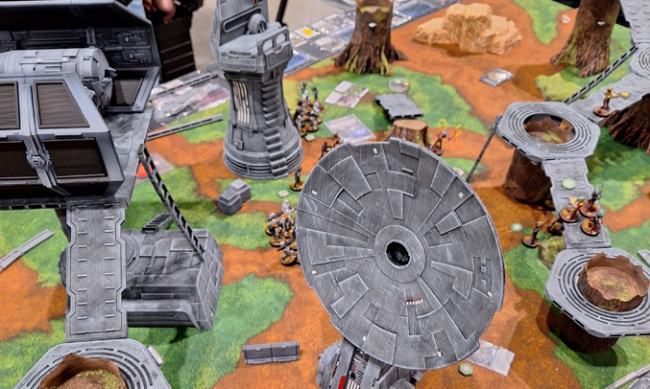In this detailed and immersive image, we see a meticulously crafted model set resembling a scene straight out of a fantasy or sci-fi world, potentially inspired by Star Wars. The landscape features a brown field with scattered patches of green grass and numerous cut-off tree stumps. Wisps of orange dirt add to the alien terrain, augmenting the setting's rugged aesthetic. Surrounding the tree stumps are gray plastic platforms that wrap around the bases, connected by small bridges, evoking a futuristic ambiance.

At the heart of the model is a large, gray plastic disc, reminiscent of a satellite dish, grounded by steel-like structures laden with intricate designs, suggestive of a high-tech environment. Fencing and barricades dot the landscape, enhancing the sense of a strategically game-oriented scene. To the left, a prominent ladder ascends to a tall platform, adorned with contrasting shades of gray plastic that mimic industrial machinery. 

The game board-like setup features inch-tall figurines with brown bases scattered across the platforms and bridges, hinting at a dynamic tabletop gaming scenario. These figures appear to be navigated by players around the table, engaging in a campaign akin to Dungeons and Dragons. The realistic details – from satellite-like structures and space vehicles to the vivid portrayal of varied terrain – convey a vivid, interactive narrative where every piece of the model contributes to an intricate and fascinating fantasy world.